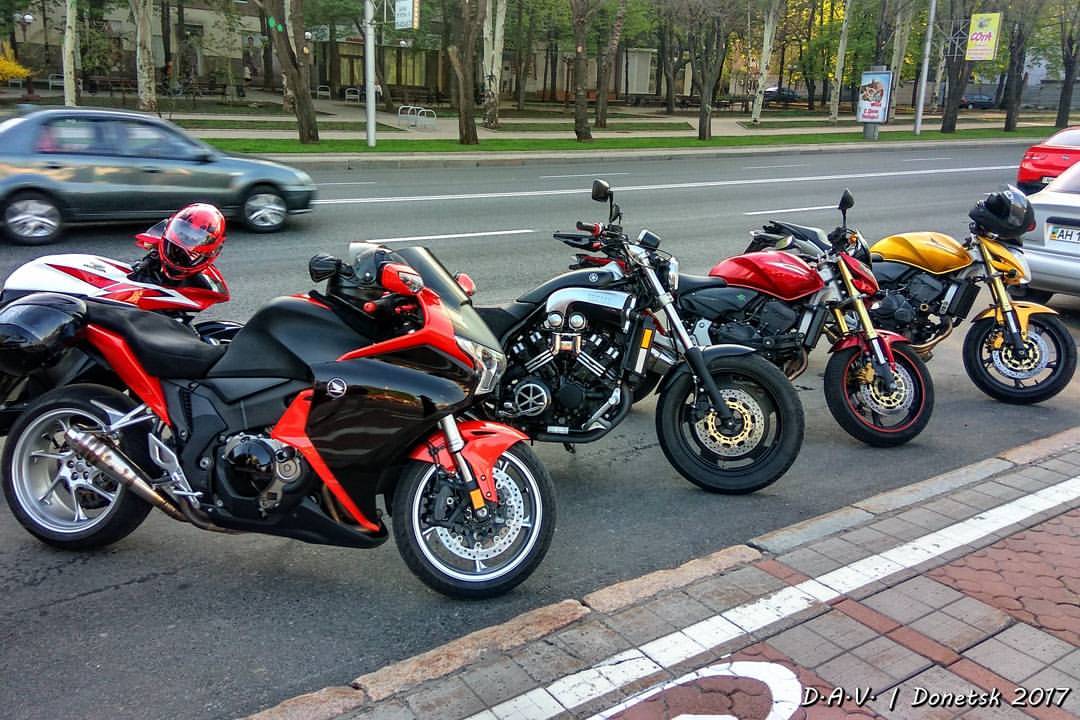The image, taken outdoors, showcases a distinctive lineup of four large motorcycles parked diagonally on a city street curb. From left to right, the motorcycles are arranged with their front wheels pointed towards the curb and the rear ends facing towards the street. The first motorcycle, adorned in red with black accents, has a helmet sticking out of its seat. The second motorcycle features a sleek black and silver chrome design. The third motorcycle is a blend of red, yellow, and black, with notable red accents. The fourth and final motorcycle in the lineup is yellow with black accents, and it sports an all-black helmet placed at the front. Behind the motorcycles, a car—appearing dark green or black in color—is seen driving by, while the back of a bright red car is also visible further down the road. The city street itself features white lines running along its length, and across the street, a park area with lush green trees, grass, and sidewalks can be observed. The bottom right corner of the image displays the lettering "DAV / Dawn of Tusk 2017." In the foreground, a gray and red brick path with an intricate design adds a touch of texture to the setting.